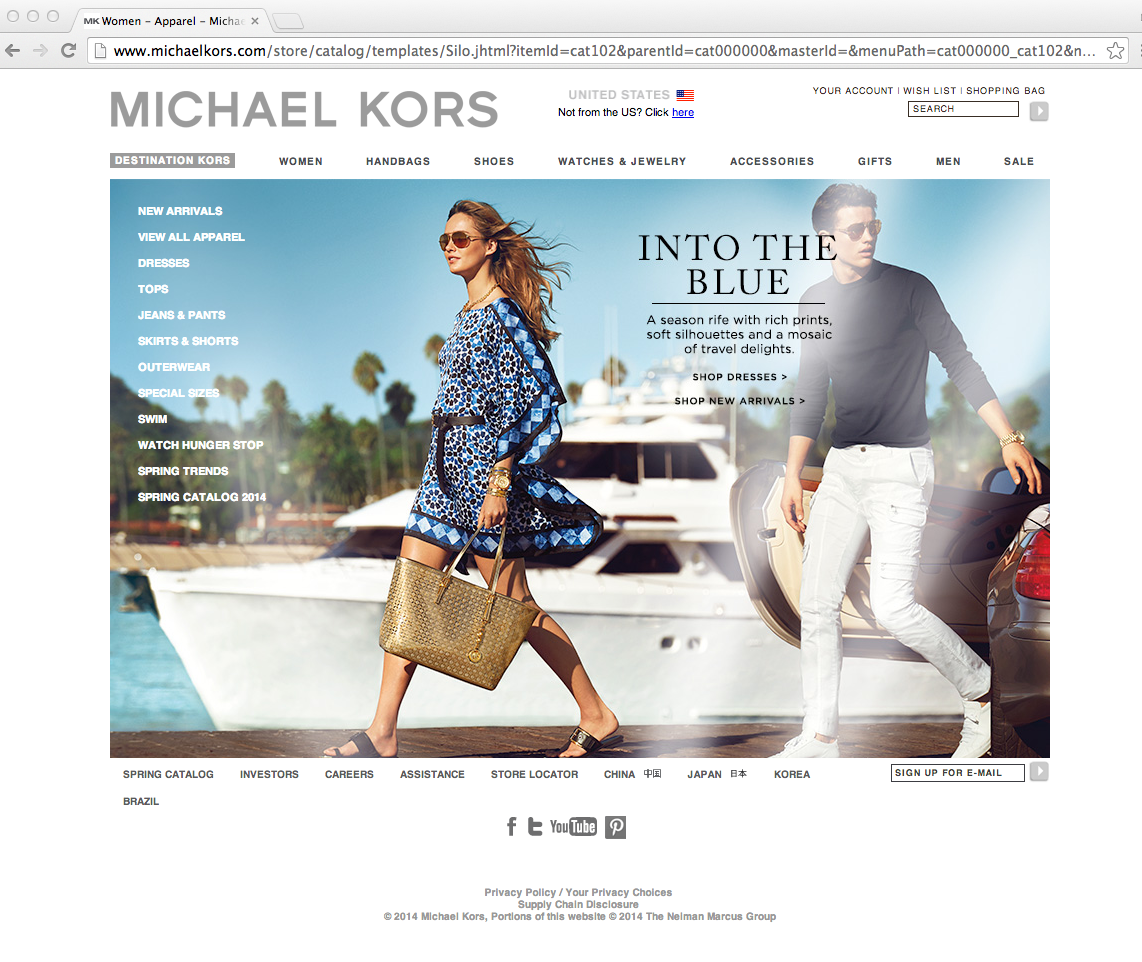The webpage features an advertisement from Michael Kors. At the top, the URL "MichaelKors.com" is entered in the search bar, leading to a well-crafted screenshot of the site.

In the upper left corner, the Michael Kors logo is prominently displayed. The browser tab reads "Women Apparel Michael." Situated in the top right corner of the page, a message on a white background reads "United States - Not from the US? Click here" in blue text. The header also includes icons for "Your Account" and a search bar.

Beneath the header is a navigation bar offering several categories: Destination Kors, Women, Handbags, Shoes, Watches and Jewelry, Accessories, Gifts, Men, and Sale.

The central image features a stylish man and woman walking away from a luxurious sports car. The woman is adorned in a short, flowy dress and carries a signature Michael Kors tote, noticeable by the metallic MK insignia. She has long brown hair and wears sunglasses. The man beside her also sports sunglasses, and is dressed in white pants, white shoes, and a gray long-sleeve top. Behind them, the left headlight of the sports car is visible as well as a large boat anchored in the background.

To the left of the image, a vertical menu offers additional categories such as New Arrivals and View Fall Apparel. In the bottom right corner of the page, an option to sign up for email updates is available.